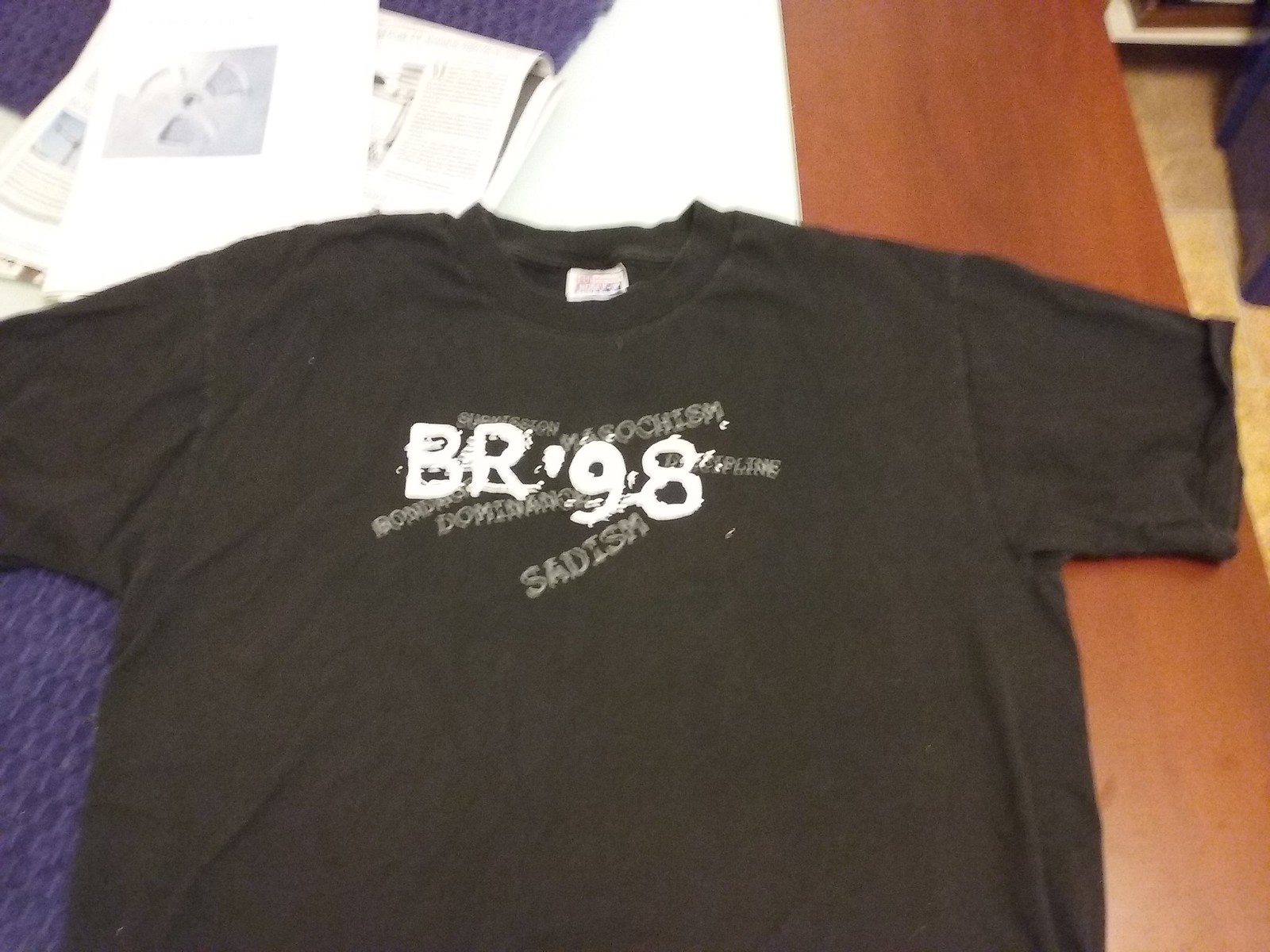A black t-shirt is laid out on a dark brown wooden table. The shirt features the text "BR 98" prominently displayed, accompanied by the words "Sadism Dominance Masochism." The context or significance of "BR" and "98" remains unclear. The table is partially cluttered, with some papers scattered underneath the shirt, particularly in the top left corner of the image. The overall ambiance of the picture conveys a somewhat dark and enigmatic theme.